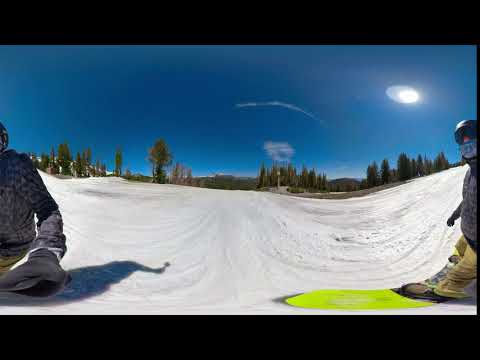The image depicts two snowboarders on a snowy slope under a bright blue sky. The snowboarder in the forefront stands confidently on a lime green snowboard, sporting yellow pants, a blue jacket, a helmet, and ski goggles with a bandana covering their mouth. This person seems to be holding a camera in their left hand, suggesting a 360-degree panoramic view as indicated by the distortion lines in the image. Beside them, another snowboarder is partially visible on the left side of the photo, seated on a black snowboard and clad in a purple and yellow sweatshirt. The vivid scene is bathed in sunlight, with the sun positioned in the top right corner, accentuating the snow-covered slope. In the backdrop, there is a range of distant mountains and sparse green trees dotting the snowy landscape, along with a single cloud and a jet stream painting the otherwise clear sky. Additionally, some poles and other structures are faintly visible, adding depth to the expansive wintery setting.